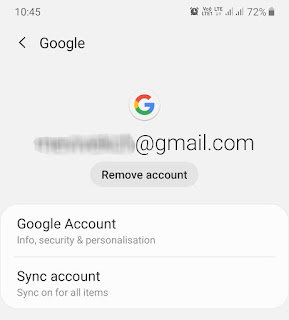The image features a light gray background with a light gray border. In the top-left corner, the time is displayed as 10:45, while the top-right corner showcases several icons, including a signal strength indicator with three out of four bars, and a battery life showing 72%. Below these icons, towards the left, there's a black arrow pointing left, accompanied by the word "Google" on the right side.

Centrally aligned, there is a white circle with the rainbow-colored Google 'G' symbol, which prominently stands out in the center. Directly below this, another centered line of text displays an email address in the format "xxxxx@gmail.com," but the actual address is blurred out.

Beneath the email address, there's a slightly darker gray oblong button with the text "Remove Account" written in black. Following this button, a white rectangular section can be seen. At the top of this section, "Google Account" is written in black text, followed by "Info, security, and personalization" in gray text.

Below this description, a horizontal light gray line divides the sections. Finally, underneath the line, "Sync Account" is written in black text, with "Sync on for all items" written in gray text just below it.